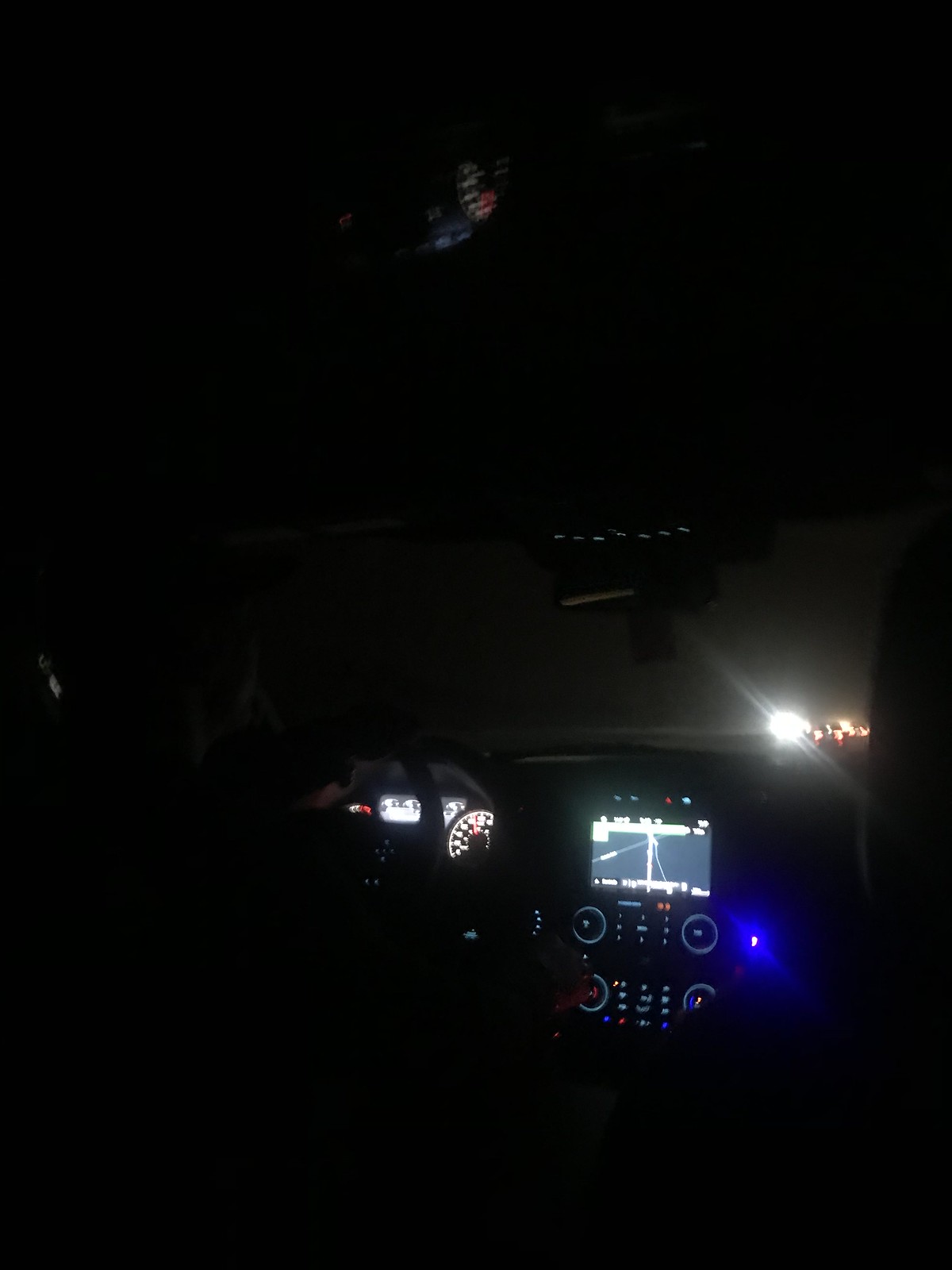Captured against a pitch-black night sky, this image subtly features a faint, possibly reflective, red and blue light in the upper-middle section. The viewer's perspective is from a car's interior, revealing a detailed view of the dashboard. Centered is a GPS unit flanked by two control panels, each adorned with a large central knob and flanked by smaller buttons. Beneath these panels, another set of controls is faintly illuminated by a soft blue light. On the right, the white speedometer and additional instrument panels are clearly visible, along with a partial view of the steering wheel. Ahead, the headlights of oncoming traffic pierce through the darkness, adding depth and context to the scene.